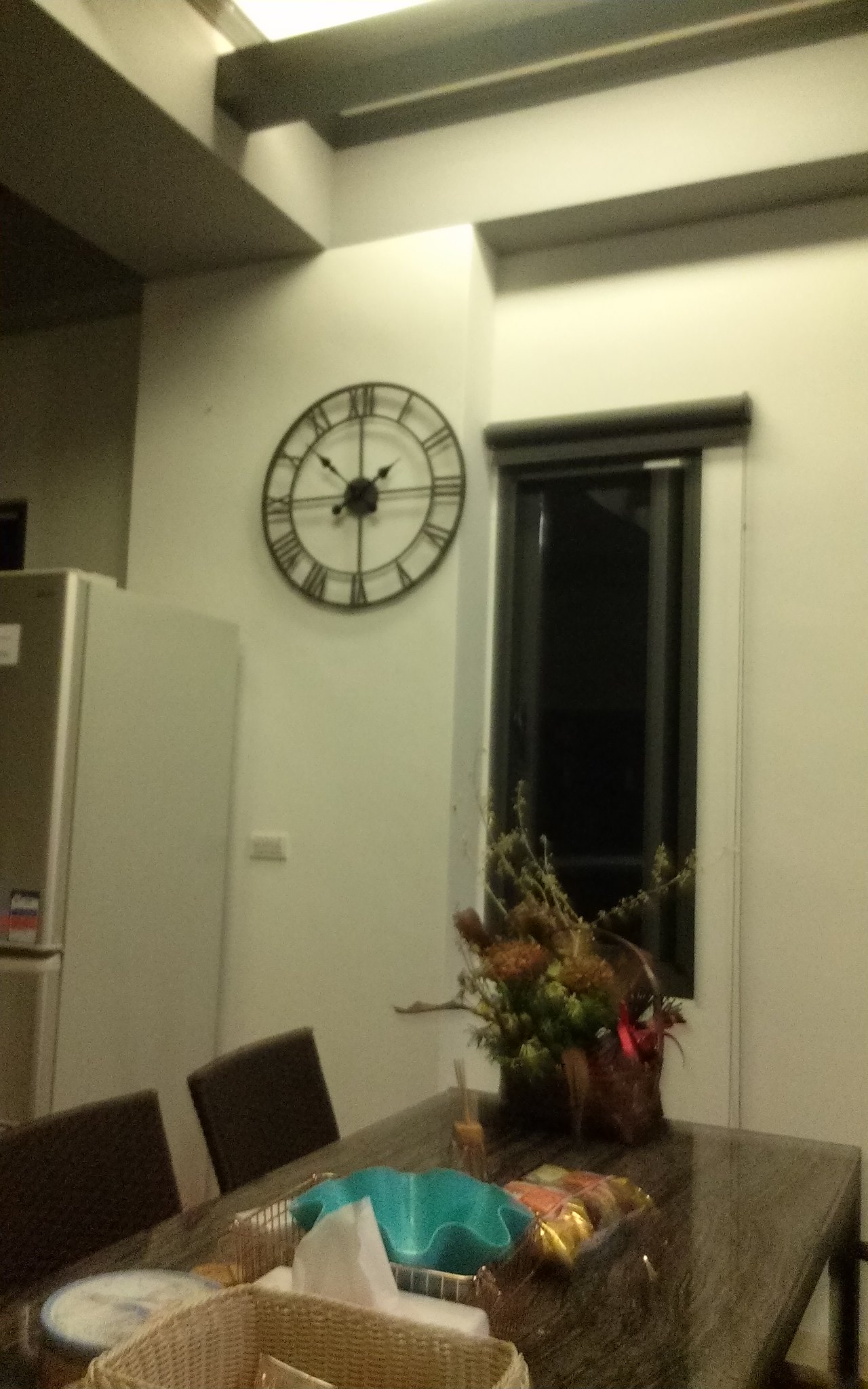The photograph captures the inviting interior of a home's dining area, centered around a dark, glossy wooden table that reveals a rich wood grain. The table is accompanied by two brown chairs positioned on its left side. At the heart of the tabletop sits a basket, a single clamshell-shaped blue bowl, and a vase containing a flower arrangement that appears to be wilted. A wall clock with an ornate, cutout metal design and Roman numerals, displaying the time as 1:52, hangs between a door with a window and a sleek, silver refrigerator. The door seems to lead outside, adding a touch of natural light to the cozy breakfast nook.